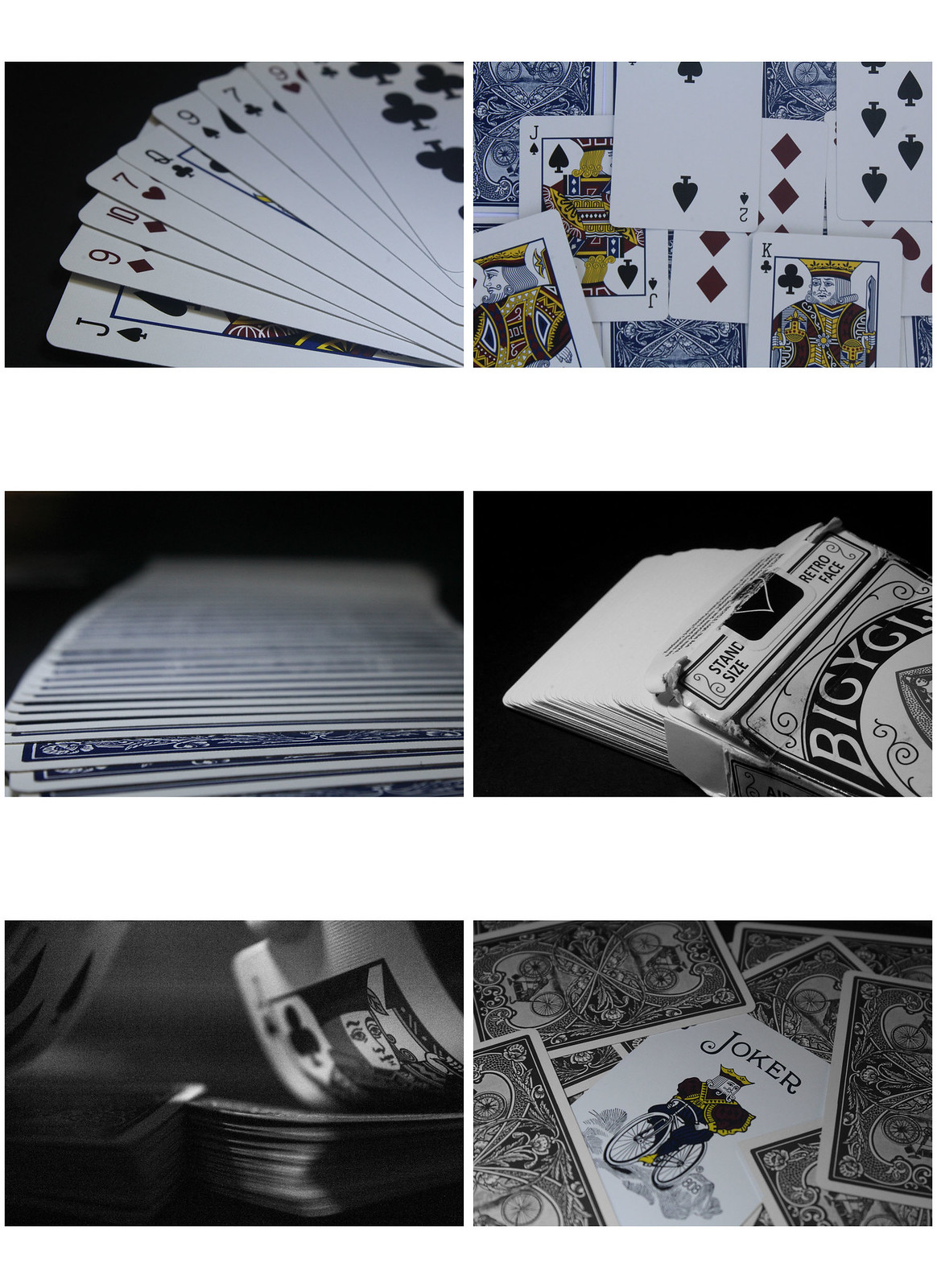This image is a screenshot displaying a collection of various photographs of playing cards, organized into three rows with two images per row. Each image is set against a simple white background, while the cards within these photographs are placed against different backdrops.

- In the top-left image of the first row, a sequence of cards is neatly arranged side by side on a black background, showing only their top-left corners which display the suit and value. Examples include the nine of diamonds and the ten of hearts, all presented in black card designs.

- The top-right image features a different arrangement where cards are haphazardly scattered, overlapping each other against a blue backdrop.

- The second row's left image mirrors the top-left one in arrangement but shows the cards face-down, making their identities unknown.

- The second row's right image is black and white, illustrating the case of the cards with several of them flying out of it.

- The black and white theme continues in the bottom-left image, which depicts a jack card dramatically bent or in mid-flip.

- Finally, the bottom-right image showcases a joker card prominently placed face-up among other face-down cards, creating a striking contrast.

Each photograph within this screenshot captures a different aspect or arrangement of playing cards, emphasizing varied visual styles and backgrounds.